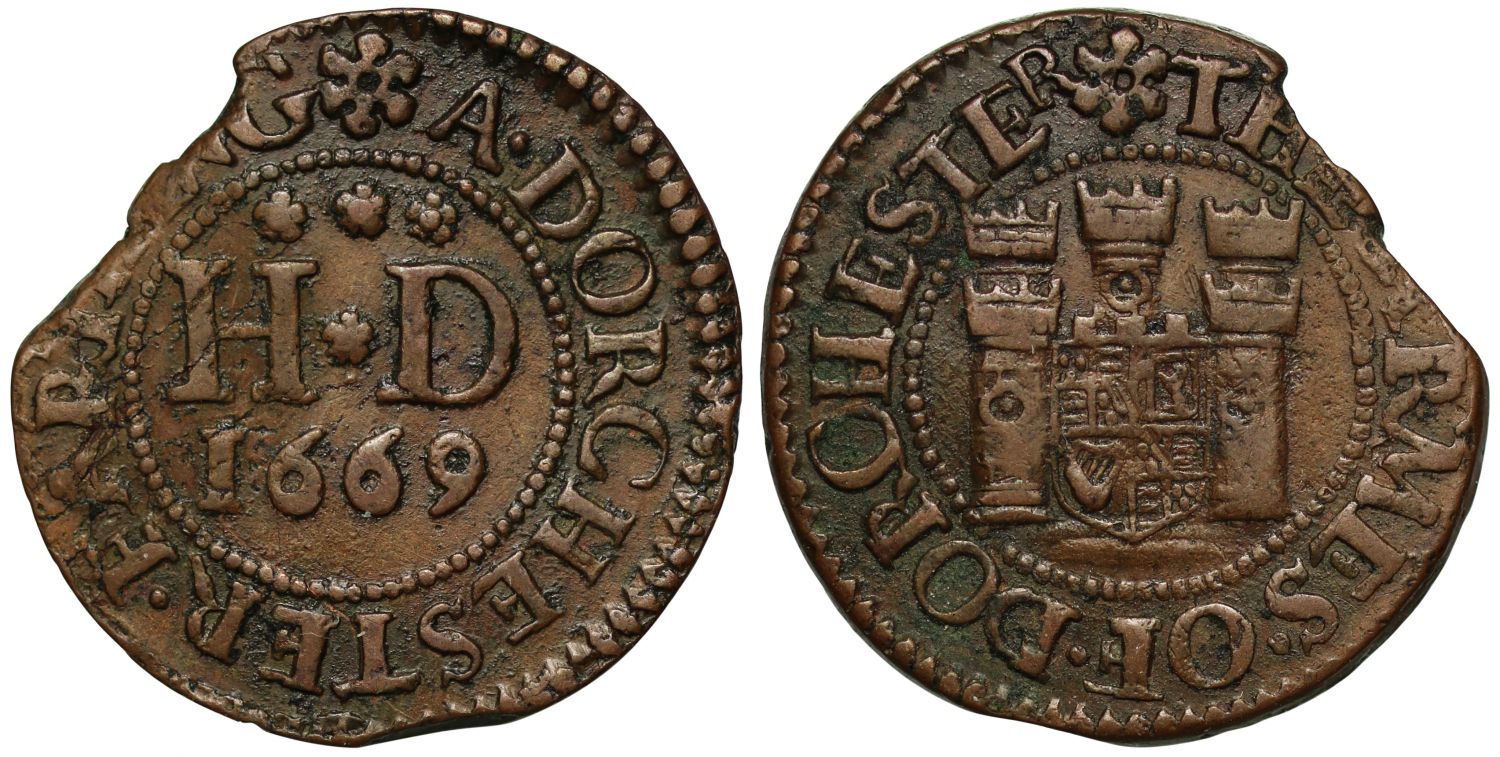The photograph features the front and back of an old, weathered coin, predominantly brown with black accents, against a white background. Both sides of the coin are chipped, giving them an irregular, non-uniform shape. The coin appears handmade, and this is evident from its texture and the varying thickness around the edges. The side on the left displays the letters "HD 1669" prominently in the center, surrounded by a beaded circle and an outer ring of letters that partially spell "DORCHESTER." The right side, likely the reverse, showcases a detailed engraving of a castle in the middle, encircled by the remaining fragments of the inscription. The coin's intricate beading and partially obscured inscriptions suggest it holds significant historical value and artistic craftsmanship.